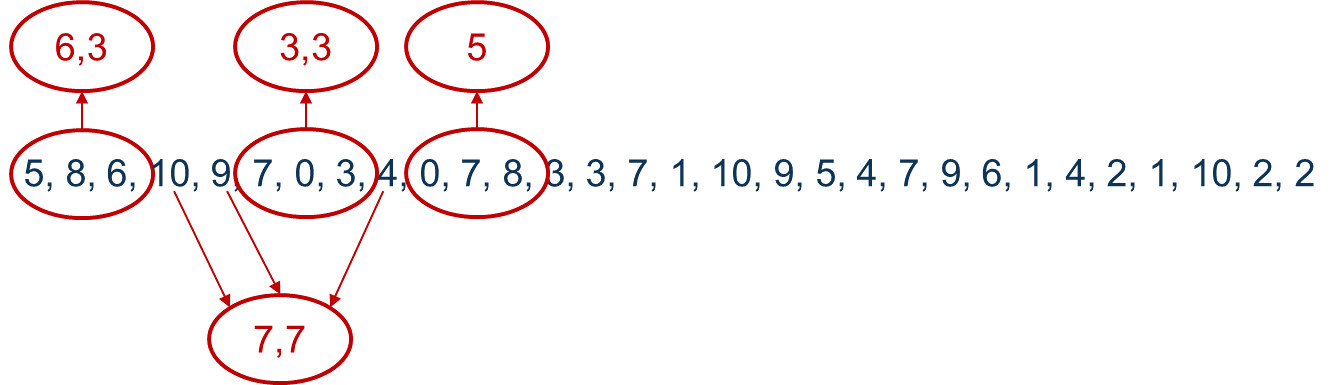In the image set against a white background, the top left corner features a red circle containing "6,3." To its immediate right, there are two more red circles; the first one encloses "3,3" and the second contains the number "5." Below these, the number "586" is presented in black, circled in red, with an arrow pointing upwards. Adjacent to this is "109," also in black, with an arrow pointing diagonally downwards towards a red circle that holds "7,7." Further below, the sequence "7,0,3," circled in red, has an arrow pointing upwards. Near the bottom, the number "4" in black is accompanied by a red arrow pointing diagonally downwards. To the right of this, "0,7,8" is circled in red with an arrow directed upwards. Following this is an extensive series of numbers in black, ".3,3,7,1,10,10,9,5,4,7,9,6,1,4,2,1,10,2,2."